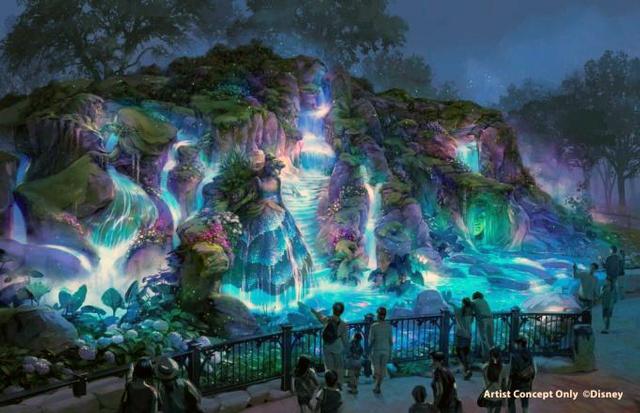This digital image, labeled "Artist Concept Only, copyright Disney," illustrates a mesmerizing nighttime scene at a Disney theme park. The focal point is an enchanting glowing blue waterfall cascading from a luminescent hillside adorned with vibrant hues of blue, green, and purple. The waterfall is surrounded by shrubbery and moss-covered rocks, with trees crowning the top of the hill. The sky is dark, speckled with stars, enhancing the nighttime ambiance. A wrought iron fence separates visitors from the breathtaking spectacle, creating a viewing walkway similar to zoo enclosures. There are 16 people captured in the scene, gazing in awe at the ethereal waterfalls with flowing water pooling at the base. Among the details, a peculiar human face can be seen within a cave on the center right side of the rock formation. The overall brightness and vivid colors of the water create a magical, dreamlike atmosphere.